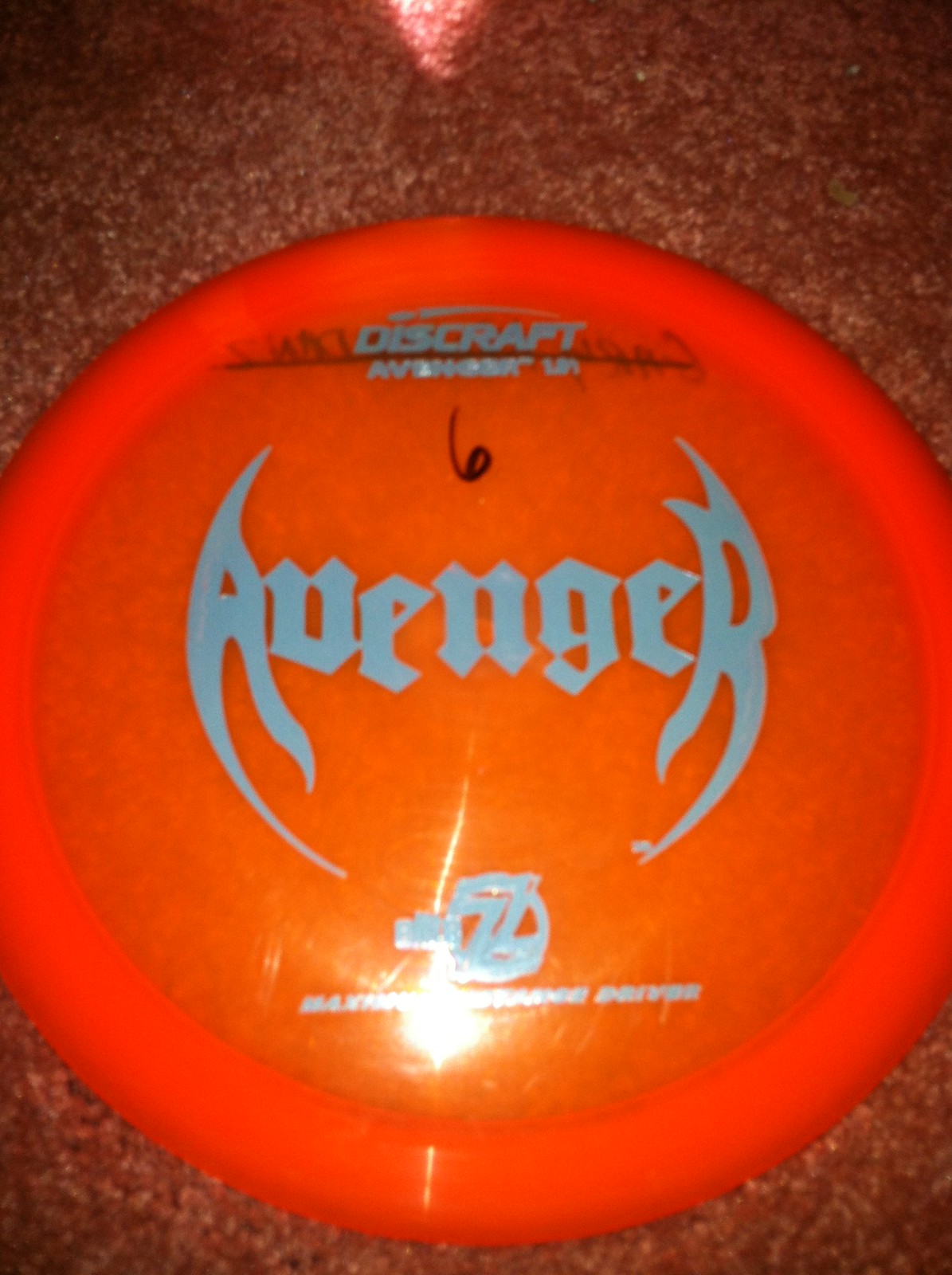The image is a close-up photograph of a well-used, reddish-orange Discraft flying disc, designed for either Frisbee golf or casual play. The disc lies on a rust-colored carpet, with the edges slightly cut off by the frame of the picture. At the top of the disc, the word "DISCRAFT" is prominently displayed in blue letters. Below this, the word "AVENGER" is printed in light blue, featuring stylized, enlarged 'A' and 'R' at the beginning and end, respectively. In the center, a black "6" is handwritten with a marker. Beneath the "AVENGER" logo, an intricate circular graphic with a "Z-Z-Z" pattern is partially obscured by a reflection of light, likely from the camera flash. The disc is flatter and thinner than typical Frisbees, indicating its design for specialized use. There are some scuffs around the edges, revealing its well-used condition.